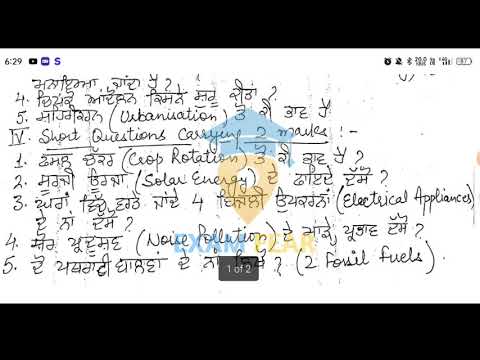The image is a detailed screenshot of a virtual whiteboard or app. The whiteboard features a diverse array of handwritten text in a black marker, including symbols, mathematical formulas, and notations in both a foreign language and English. Notable English phrases such as "crop rotation," "solar energy," "noise pollution," and "fossil fuels" are interspersed among the text. The layout indicates a structured lesson plan or notes, possibly including short questions and a numbering system. The image also contains a virtual interface with a few navigational icons on the top right, including a battery symbol, an alarm symbol, and a silence icon, while the top left displays a digital clock and some notification icons. There is a faint logo in the background featuring a blue graduation cap and a brown head. At the bottom center, a black box indicates the text "1 of 2." The overall style is that of an informational graphic, captured in a horizontal landscape orientation.